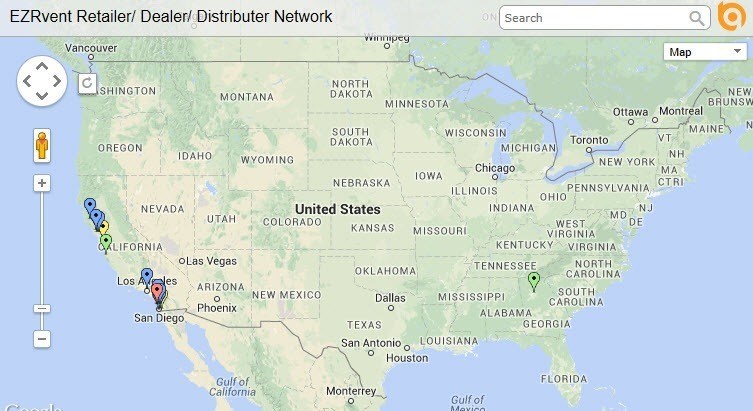This image features a detailed map of the United States with several notable elements. At the top of the image, there is a gray border containing black text on the left that reads "EZREVENT," with "E-Z-R" in uppercase and "vent" in lowercase. Following this, the text describes "Retailer / Dealer / Distributor Network." On the far-right side of the border, there is a search box.

An orange logo resembling a bullet point is also present near the top. The map itself shows not only the United States but also parts of Canada, including cities like Vancouver, Winnipeg, Toronto, Ottawa, and Montreal.

To the left of the map, there is a box labeled "Map" with a dropdown arrow, a direction icon, and a person icon that can be placed on the map. Additionally, there is a slider that allows users to zoom in or out, ranging from negative to positive.

In the main body of the image, the map of the United States is populated with multiple location icons, all concentrated in California. Specifically, there are around ten location markers situated in areas such as Los Angeles, San Diego, and Northern California. The map also displays major bodies of water, including the Gulf of Mexico, and the Atlantic and Pacific Oceans.